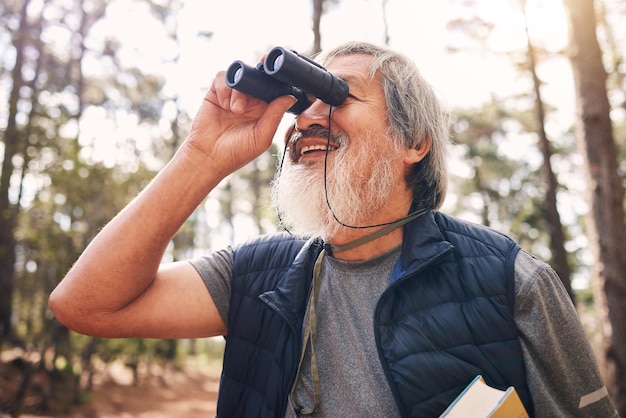In this detailed close-up image, we see an individual standing in a forest setting, gazing through a pair of black binoculars. The person, who has a mostly white beard and gray hair that slightly extends past the ears, is wearing a light gray shirt beneath a dark blue vest. The binoculars are held up by the left hand while the person's face is lit up with a smile, revealing the top row of teeth. The binoculars are suspended from a gray case hanging around the neck, with thin black straps visible. 

At the bottom of the image, there's a glimpse of an open book with white pages adorned with several blue lines, and a light brown cover peeking out slightly. The background is an out-of-focus forest with numerous trees and lush green leaves, through which bright white light filters, adding a soft, natural illumination to the scene.